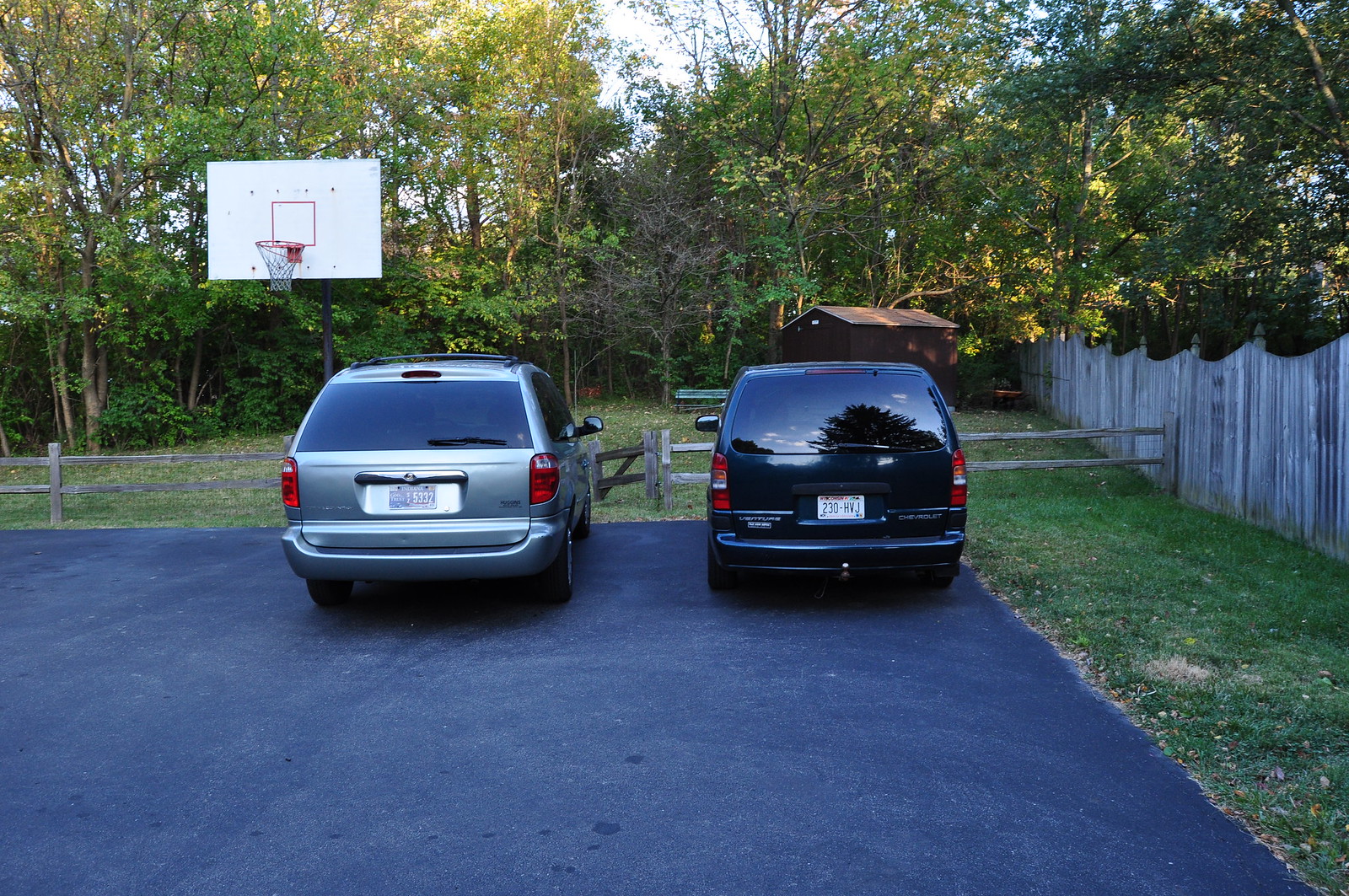This image depicts a backyard or yard area converted into a paved parking lot, bordered by regions of green grass. The parking area is enclosed by a combination of fences: a farm-like wooden fence running horizontally from left to right and a taller, vertical slat privacy fence lining the right side. In the background, a dense array of tall, green-leafed trees creates a natural woodland backdrop, situated in front of which is a dark brown wooden shed or structure. The yard features two parked minivans, one silver on the left and the other a dark blue or possibly dark green on the right. Adjacent to the silver minivan, there is a basketball goal post set up on the left side of the image, adding an element of recreational use to the area. The pavement of the yard suggests it's a multifunctional space, blending a makeshift sports area with a practical parking lot.